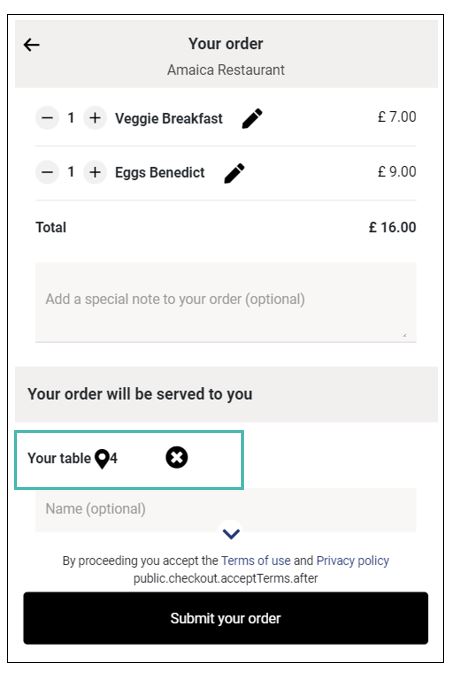This is an image of a restaurant order displayed on a rectangular screen. At the top center, the header "Your Order" is prominently written in bold black text. Beneath this, in a lighter black font, it is indicated that the order is from "AMAIKA" restaurant, with the name spelled as "A-M-A-I-C-A." 

The first item listed is "1 Veggie Breakfast" followed by a pencil icon, and it is priced at £7.00. Underneath this, the second item, "1 Eggs Benedict," also features a pencil icon and is priced at €9.00. The total cost of the order is summed up as €16.00.

Further down, there is a note stating, "Your order will be served to you." Below this, the text indicates "Your table: 4," and it ends with an optional field for the name.